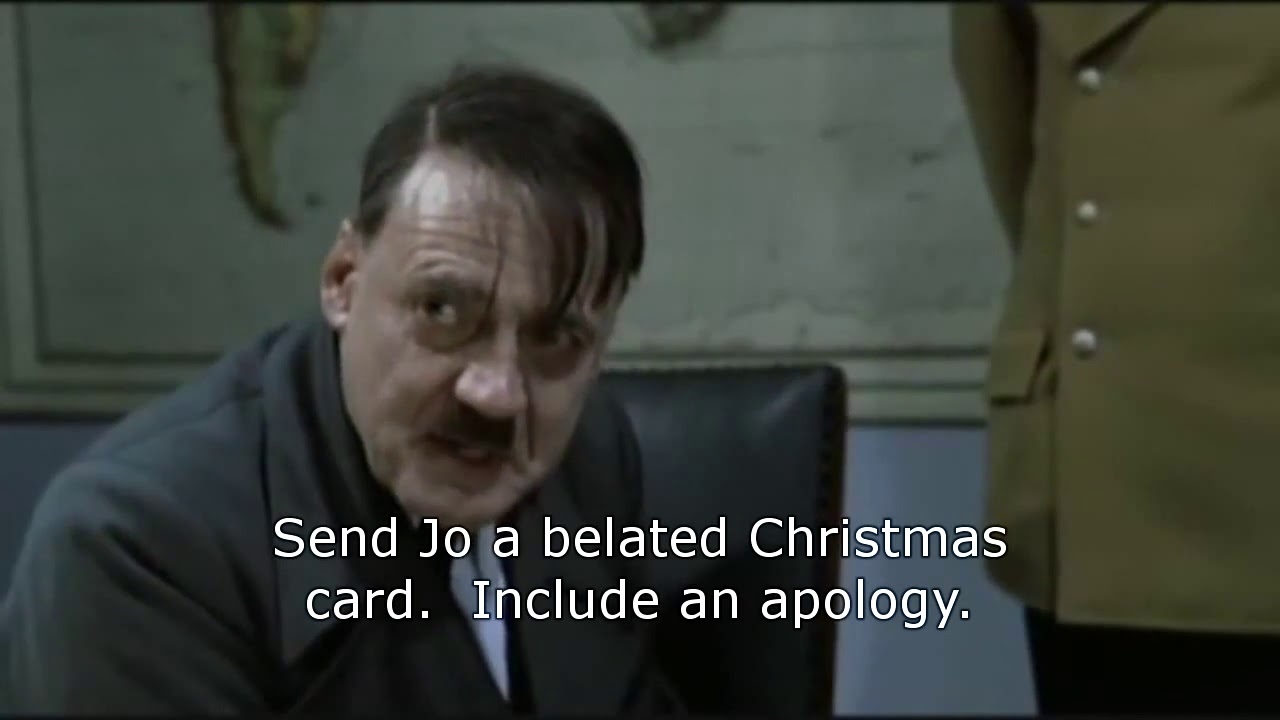This image appears to be a still from a movie scene, depicting an actor resembling Adolf Hitler. The actor, identifiable by his dark hair and signature skinny mustache, is seated in a black chair with his head down and shoulders slouched. His hair partially covers his face, and he is dressed in a black suit paired with a blue tie. Adjacent to him stands another man, dressed in an olive-green, possibly military-style jacket with three distinct silver buttons and black pants. The map behind them on the blue wall features green and yellow details, likely representing different regions. At the bottom of the image, in white letters, it reads, "Send Joe a belated Christmas card. Include an apology."